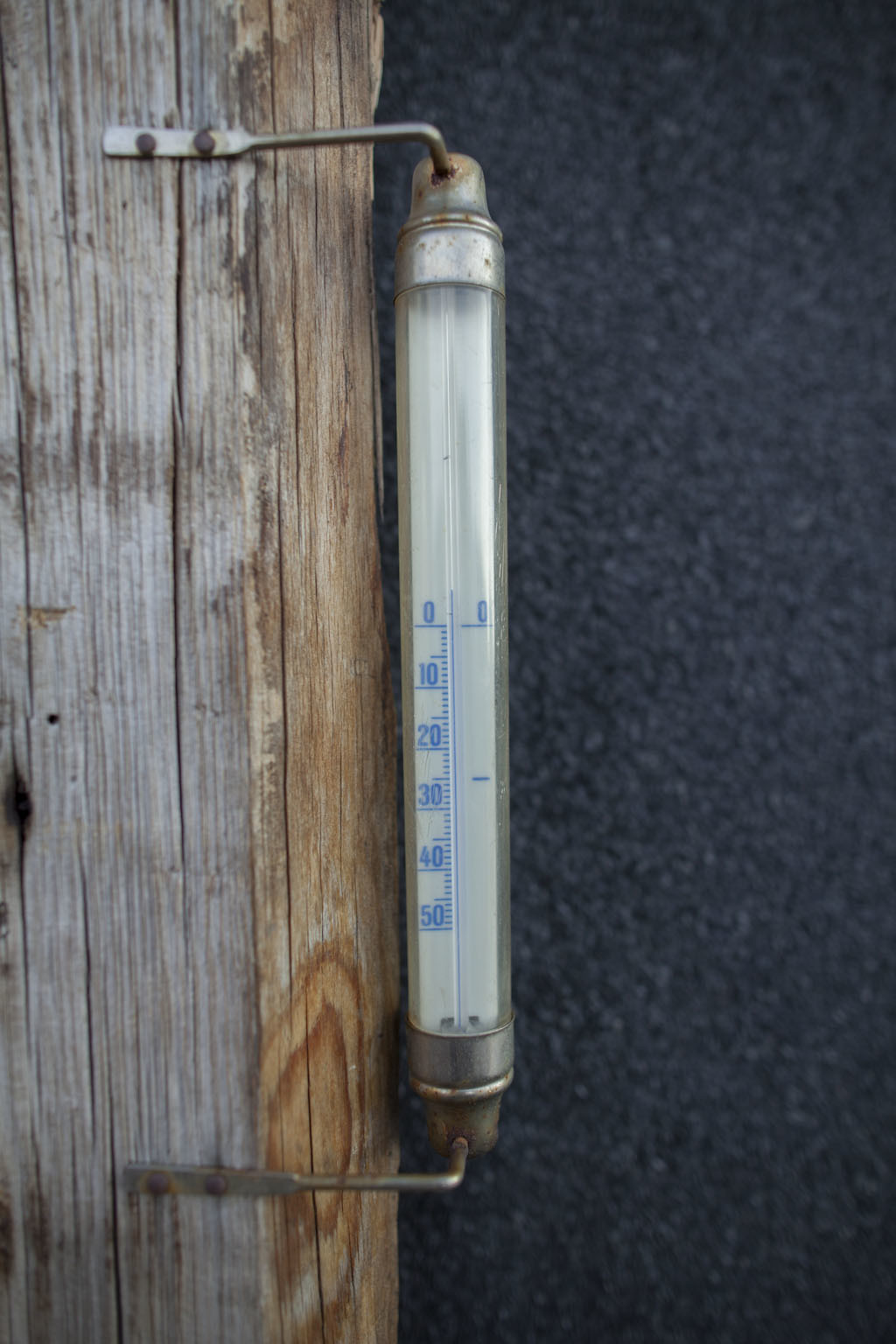This photograph captures a thermometer designed to measure extremely cold temperatures. The thermometer is housed in a clear glass tube which encases a white background with numbered markings spaced at intervals of 10, ranging from 0 down to -50 degrees. The tube itself is secured with a metal cap on both its top and bottom, each featuring a small arm. These arms are screwed into a sturdy wooden post that occupies the entire left half of the image. The thermometer fluid, which appears blue, indicates the current temperature at approximately -25 degrees. The background of the photograph shows a black, pebbly surface, possibly asphalt. The thermometer's design and scale suggest it is used in very cold environments, highlighting its specialized nature.